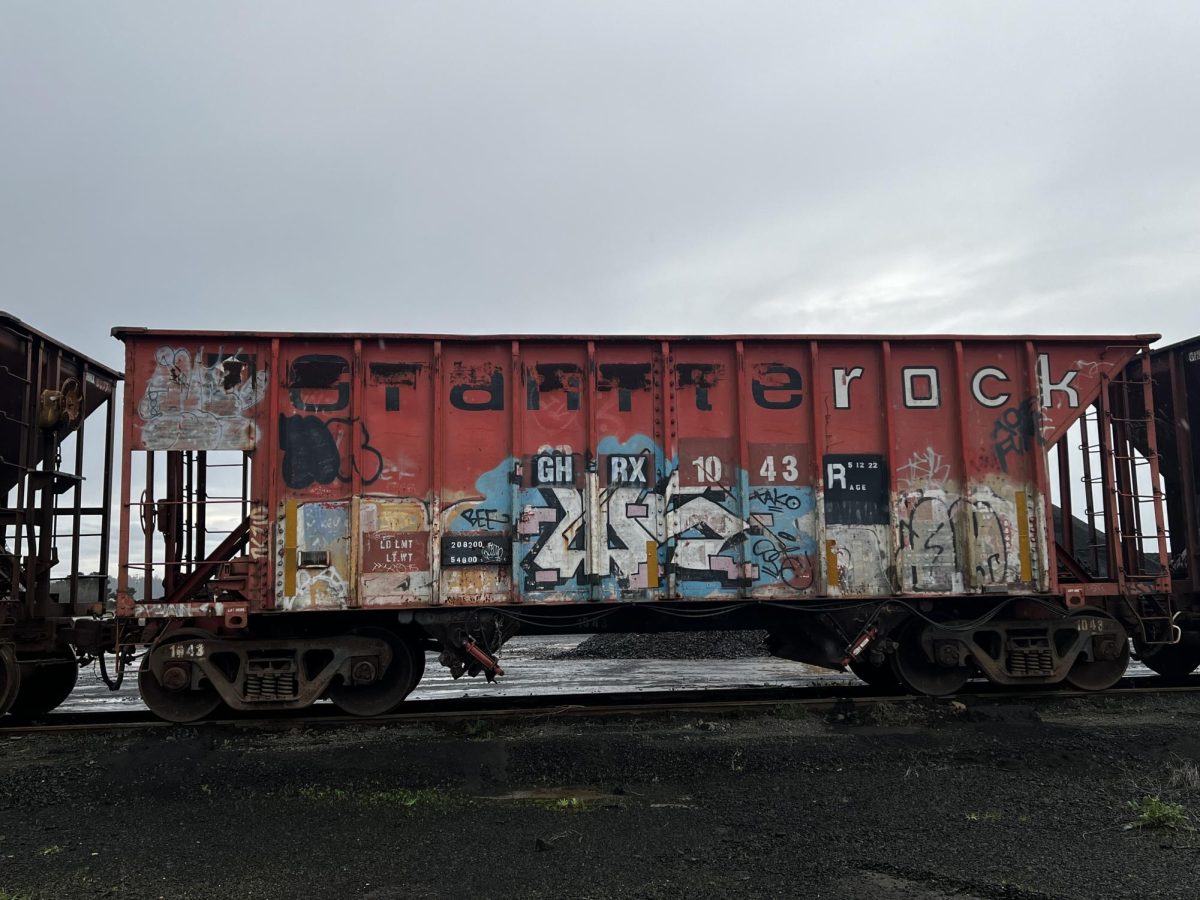The outdoor photograph depicts a weathered, brick-red freight car stationed on railroad tracks, under a predominantly gray, cloud-covered sky. The freight car, identified as GHRX1043R, exhibits significant wear and graffiti art in blue, pink, and white tones. The graffiti includes the text "S-T-A-N-T-T-E, ROCK" in white letters with a black border. Sections of the car, mainly its ends, appear hollow, suggesting it might be a coal or storage car. The ground below is characterized by dark, gravelly soil, largely devoid of vegetation, save for a small clump of green in the lower right corner. A glimpse of icy groundwater can be seen beneath the car. The scene is accented by steel wheels supporting the car on the tracks, hinting at proximity to water, likely an adjacent train yard. The overall visuals, combined with the freight car's seemingly abandoned state and the artistic graffiti, suggest the image was captured during wintertime, making it a compelling piece of self-art photography.